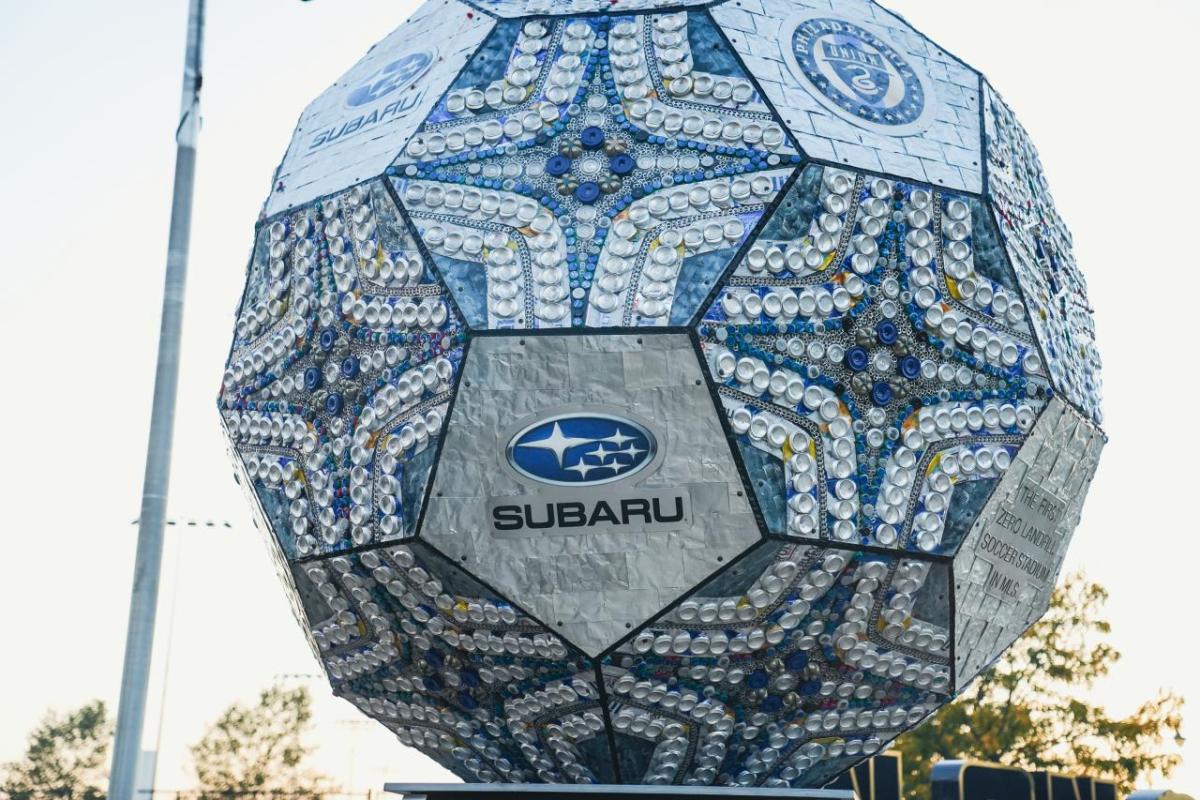The image depicts a large, outdoor sculpture resembling a soccer ball, prominently displayed outside a stadium. Each hexagonal and pentagonal panel of the ball is intricately decorated with detailed patterns and designs, featuring small, gem-like circles that form elaborate, mandala-like shapes. The pentagonal panels prominently showcase the Subaru logo—a blue oval with a constellation of six white stars—along with inscriptions such as "Subaru" and "Philadelphia." Another pentagonal panel includes the text "the first zero landfill soccer stadium in MLS." The sculpture rests on a pedestal, partially visible in the image, and is set against a backdrop of faint tree outlines and a clear, bright sky. Nearby, a flagpole or light post is also faintly visible. The color scheme of the sculpture predominantly consists of blue, white, and silver, with small touches of gold.